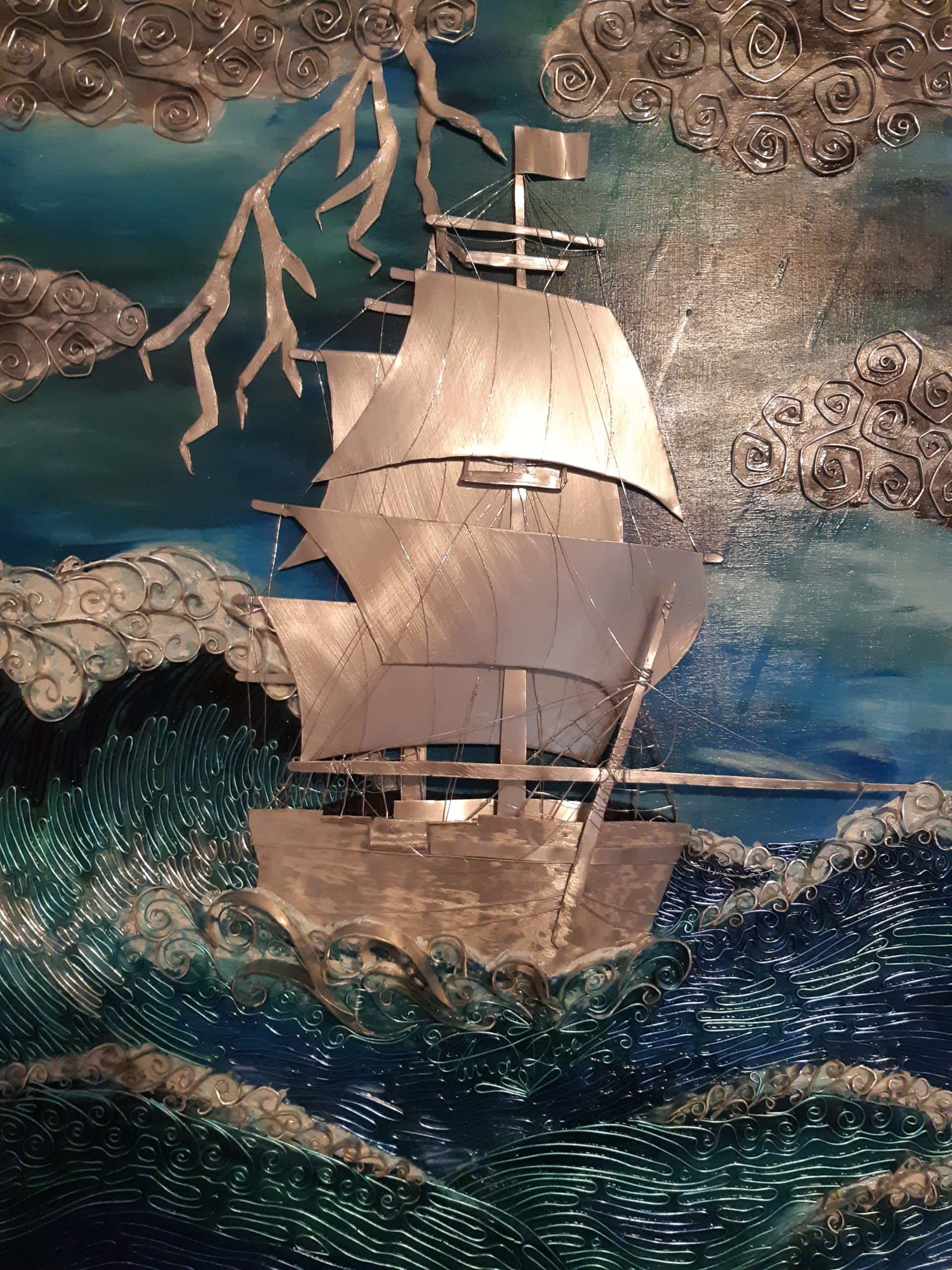The image depicts a stylized sailboat navigating choppy, decorative blue waters that appear to be crafted with watercolor or metallic elements. The sailboat, positioned front and center, features tan-colored sails and a tan hull, contrasting with the tumultuous sea below. Above, the sky is an interplay of blue hues with storm clouds in shades of grayish tan, punctuated by lightning bolts, suggesting a stormy atmosphere. The entire scene, with its rich blue and tan palette, seems almost metallic or paper-like, contributing to its artistic, surreal quality. The boat also has a visible flag atop its mast, adding a touch of realism to the creatively rendered landscape.